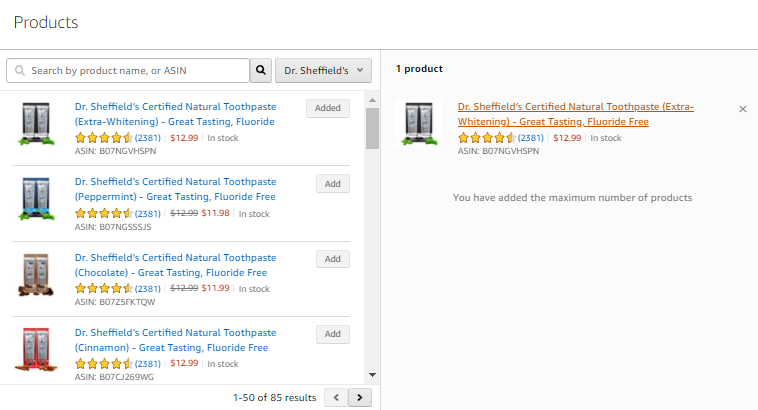This image depicts a website showcasing various products by Dr. Sheffield's. At the top left of the page, the word "Products" is prominently displayed. Directly beneath it, there's a search bar labeled "Search by product name or ASIN." At this moment, the search bar is empty, but a search icon next to it is available for initiating searches. Below the search bar, a dropdown menu is visible with the option "Dr. Sheffield's" currently selected.

The main section of the webpage features four different Dr. Sheffield's products:
1. **Dr. Sheffield's Certified Natural Toothpaste Extra Whitening** - This product boasts a four-and-a-half star rating from 2,381 reviews. It is priced at $12.99 and is listed as in stock. The ASIN for this toothpaste is B07NGVHSPN.
   
2. **Dr. Sheffield's Certified Natural Toothpaste Peppermint Flavor** - Similar to the first product, this toothpaste has a four-and-a-half star rating from 2,381 reviewers. It is priced at $11.98, is in stock, and carries the ASIN B07NG555JS.

3. **Dr. Sheffield's Certified Natural Toothpaste Chocolate** - This variant, marked down from $12.99 to $11.99, also enjoys a four-and-a-half star rating from 2,381 users. It is in stock and the ASIN is B0725FKTQW.

4. **Dr. Sheffield's Certified Natural Toothpaste Cinnamon** - This product is priced at $12.99 and is in stock. It has a four-and-a-half star rating, also from 2,381 reviews, and the ASIN is B07CJ269WG.

Additionally, at the upper right corner of the page, there is another selection highlighted as **Dr. Sheffield's Certified Natural Toothpaste Extra Whitening**. It also mentions that it has been added to the maximum number of products allowed and is available for $12.99.